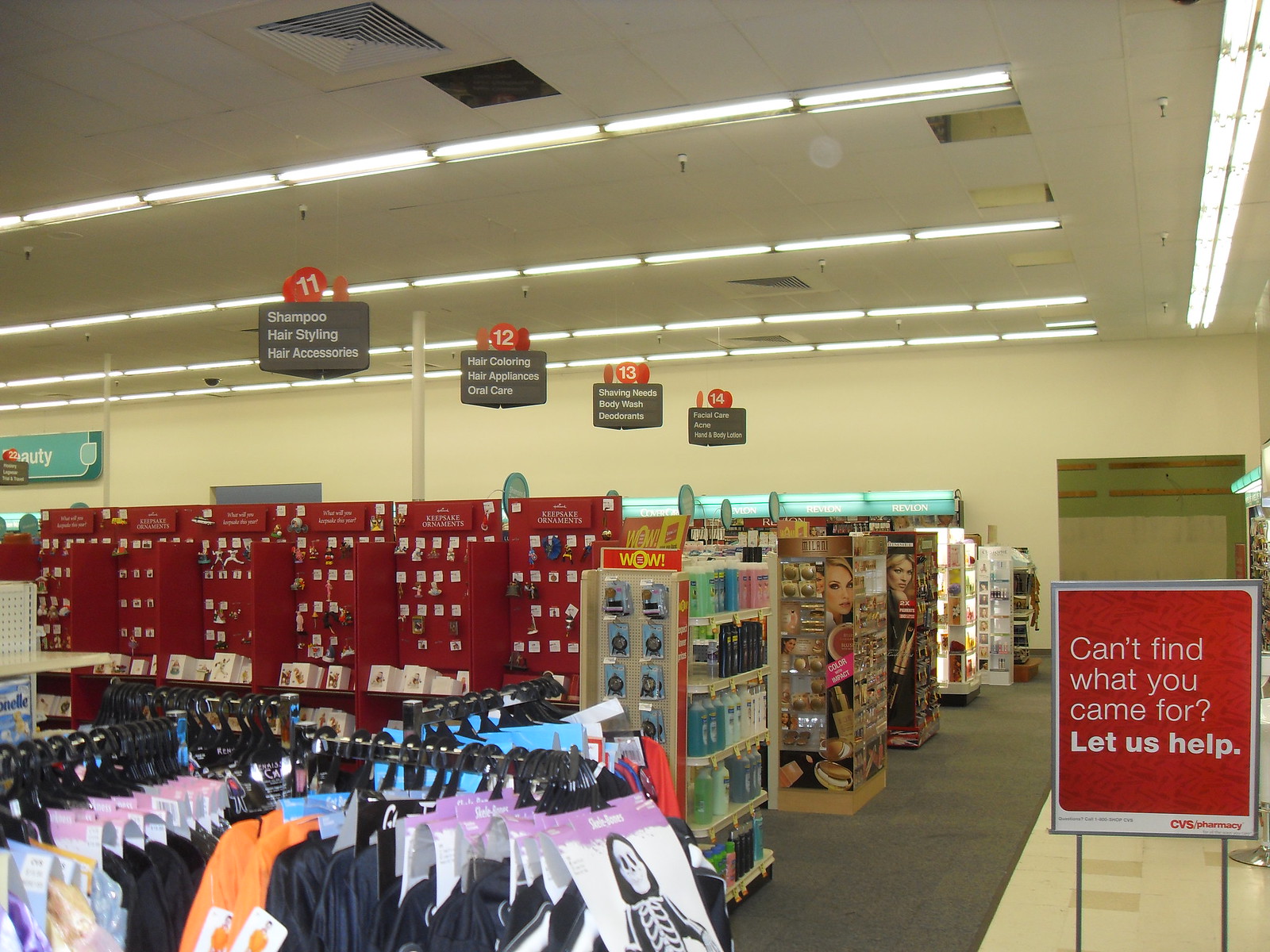This vibrant image captures the bustling interior of a CVS store. On the right-hand side, prominently displayed on a two-legged stand, is a red sign with white lettering that reads, "Can't find what you came for? Let us help," accompanied by the CVS Pharmacy logo on the bottom right. The image shows a series of aisles marked 11 through 14, well-lit by overhead lighting. Each aisle is identified by a red circular sign with white numbers and a gray rectangular label beneath it. Aisle 11 is designated for shampoo, hairstyling products, and hair accessories; aisle 12 holds hair coloring products, hair appliances, and oral care items; aisle 13 offers shaving needs, body wash, and deodorants; and aisle 14 features facial care, acne treatments, and hand and body lotion. Each sign with aisle information hangs from the ceiling for easy navigation.

In the foreground, there are racks densely packed with Halloween costumes, prominently featuring a skeleton costume, along with various black and orange outfits. The first rack showcases a collection of keepsake ornaments neatly arranged on the top shelf. Nearby, end caps are stocked with a variety of products, including Suave shampoos or body washes, and assorted Milani makeup items. Further down, the back wall is adorned with large displays for Revlon and CoverGirl cosmetics, clearly sectioned into three areas for Revlon and one for CoverGirl, providing a well-organized beauty section.